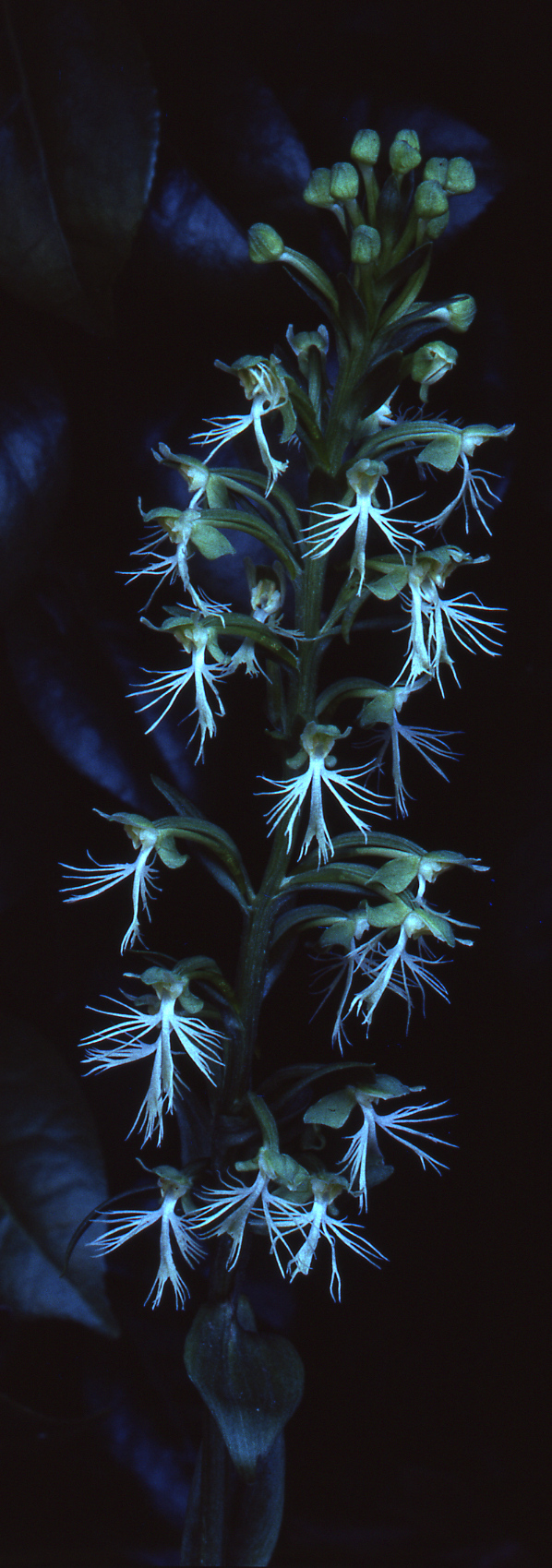The image appears to depict either a painting or a photograph, possibly taken under ultraviolet light, of a tall, vertical plant set against a pitch-black or very dark background. Along the left edge of the image, there are leaves that are purplish or dark in color, almost black. The main green stem of the plant runs through the center of the image. At the top of this stem, there are rounded green bulbs or buds, which may appear succulent-like. From these bulbs, thin, white, wispy flowers extend outward and hang down delicately from the green stems. These flowers mainly populate the edges and the sides of the image, rather than the front of the plant. In the background, there might be an outline of another plant or tree, accentuating the composition with additional, healthy-looking green leaves. The plant's appearance suggests it could be found in a warmer climate, potentially like the Southwest United States, and it does not seem to require much water, enhancing its unique, perhaps otherworldly or underwater aesthetic.